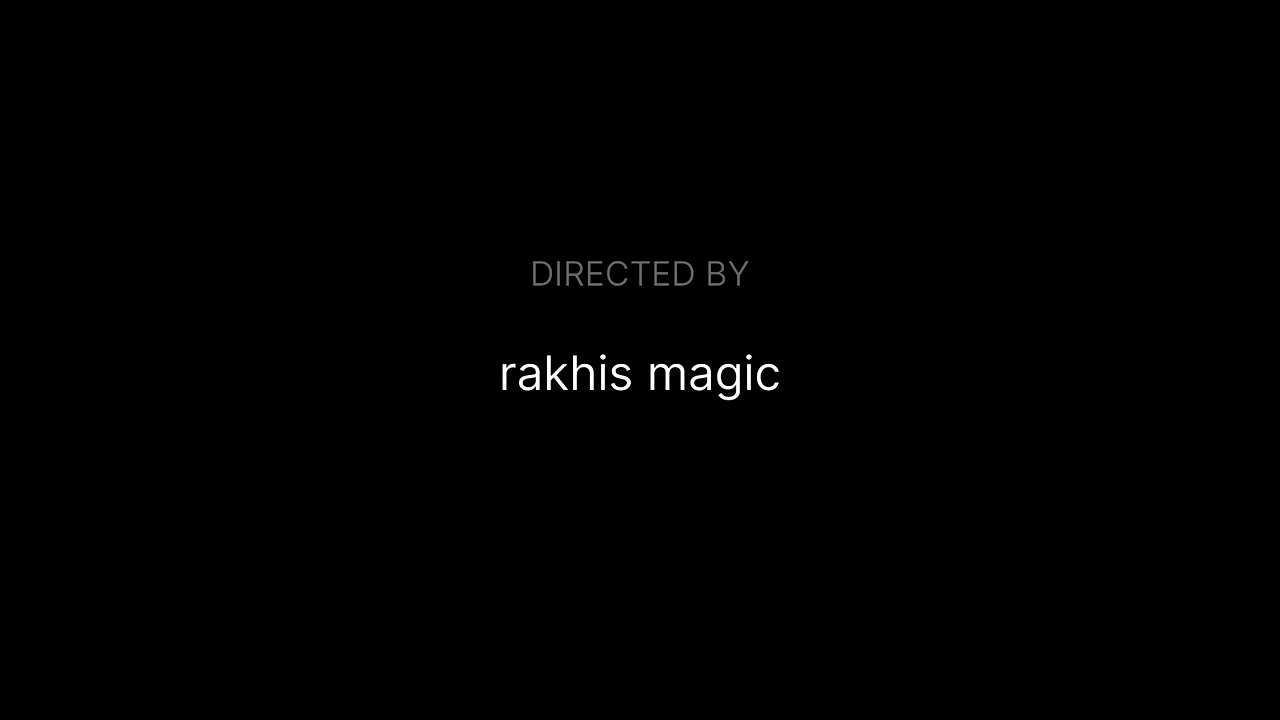The image is a simple, black, landscape-oriented rectangle. In the center, there are two rows of text. The top row has the words "DIRECTED BY" in medium gray, all caps, and a thin font. Below that, with a fair amount of space in between, the second row has the text "rakhismagic" in white, all lowercase letters. This minimalistic graphic appears to serve as a credit screen, likely indicating the director of a video or promotional material. The name "rakhismagic" is spelled R-A-K-H-I-S-M-A-G-I-C.